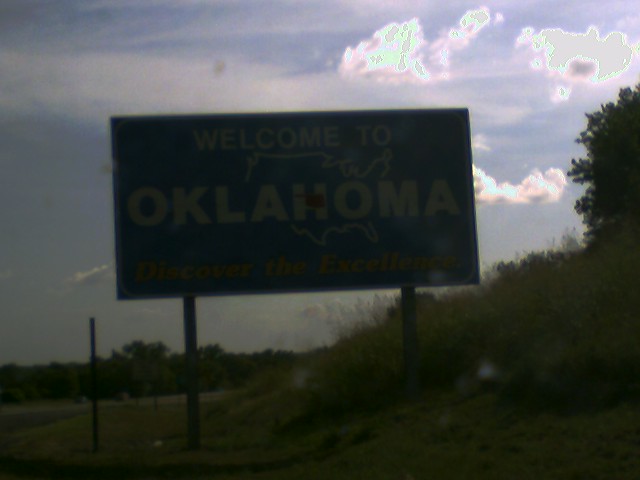This image captures a large highway sign during the early evening hours, prominently displayed on two poles—each standing on uneven ground—on the side of a road bordered by a mix of tall and short grass. The background reveals a contrast between a clear blue sky on the right and a darker, possibly overcast sky on the left. Scattered white and billowy clouds add texture to the sky, while a lone tree extends from the top right. The sign itself, primarily blue with white and yellow text, reads, "Welcome to Oklahoma" followed by the phrase "Discover the Excellence" in yellow. The sign features the outline of the state of Oklahoma. The scene is dimly lit, casting shadows that contribute to the overall moody ambiance. To the left of the sign, another black pole is visible, though its purpose remains unclear. The landscape on the right side is lush with tall grass leading down a gentle hill, while additional trees and bushes can be observed both in the background and stretching toward the center of the image. The predominant colors are green from the grass, blues and yellows from the sign, and varying shades of blue in the sky.